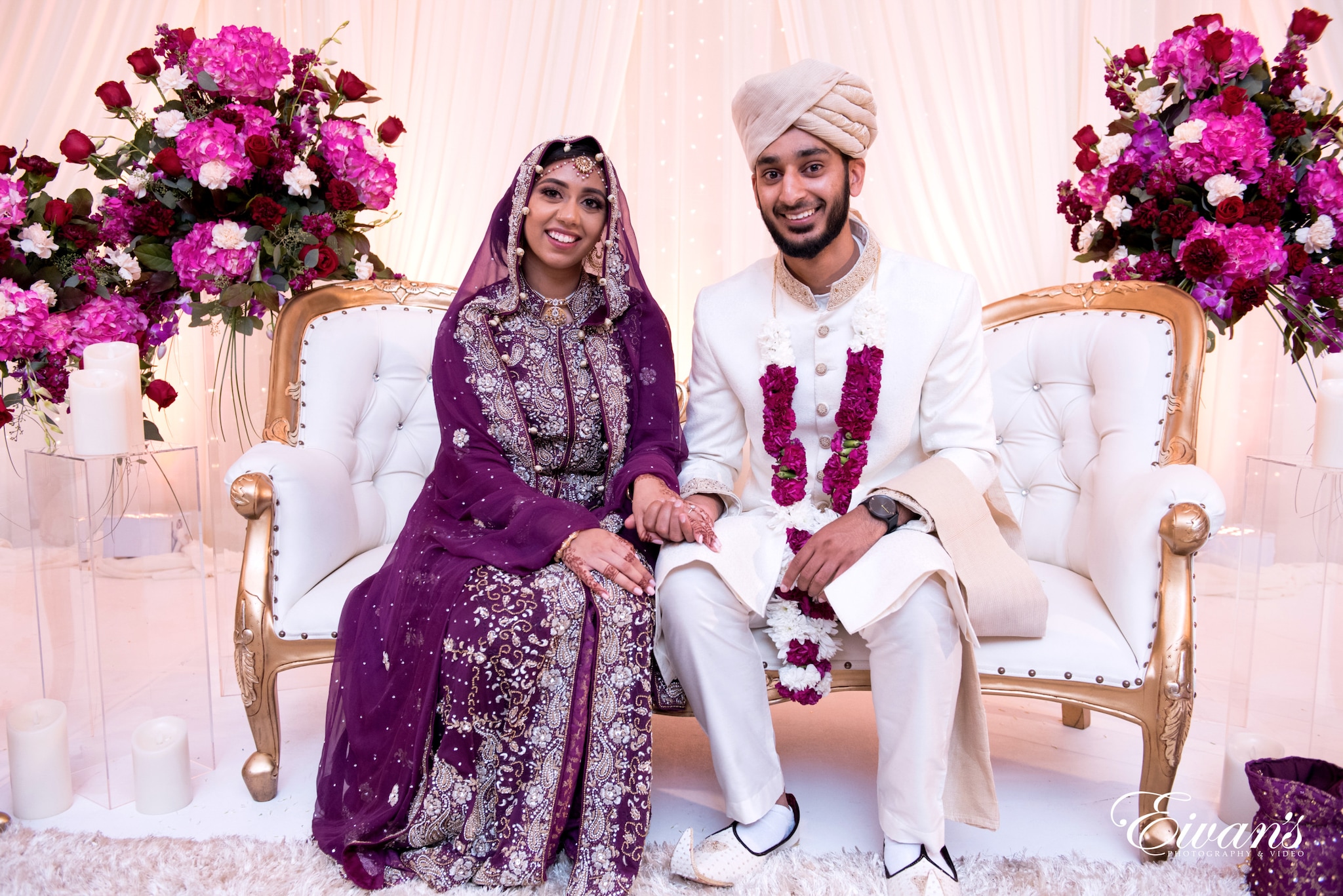In this indoor scene, a recently married Indian couple sits on an ornate white couch with gold trim, framed by lush floral arrangements and soft candlelight that hint at a lavish, possibly Bollywood-style wedding. The backdrop features elegant pink-and-white curtains, adding to the festive atmosphere. The man, positioned on the right, sports a beige turban, an intricately designed white suit with tan buttons, and white shoes with curled tips. A pink-and-white floral necklace adorns his neck, and he tenderly holds the hand of his wife. The woman on the left exudes grace in a purple dress embellished with intricate silver beading and white designs, and she drapes a purple sheer scarf over her head. She also wears jewelry, including a headpiece and rings. Their surroundings are decorated with vibrant red roses and delicate pink and white flowers arranged on clear glass tables situated on both sides of the image, complemented by white candles placed both on the tables and the floor. The setting exudes a sense of grandeur and happiness, capturing a beautiful moment in the couple's new journey together.